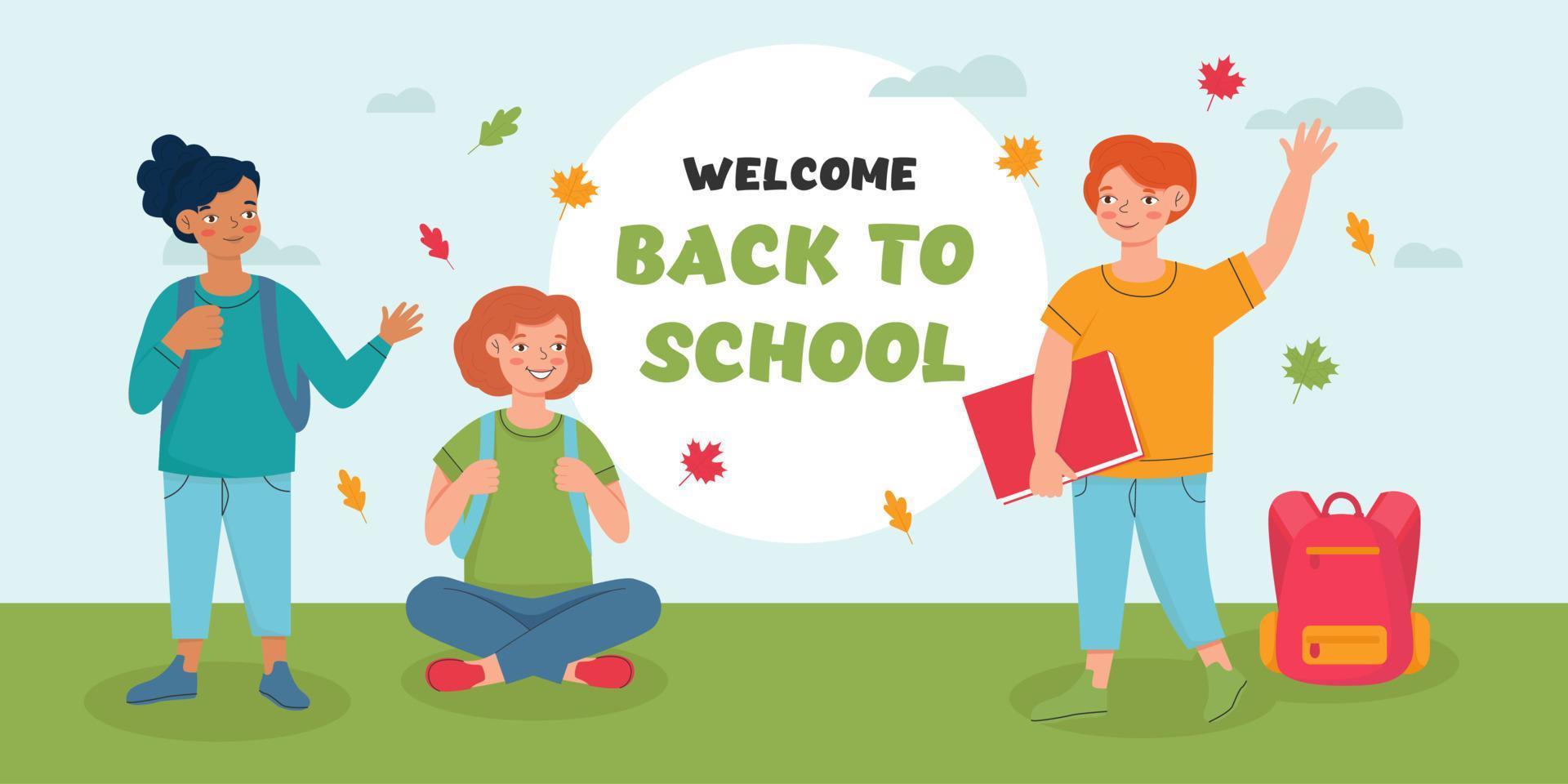In this vibrant cartoon illustration, three middle school-aged children are depicted against a cheerful backdrop of a blue sky dotted with fluffy clouds and colorful autumn leaves gently falling. The scene is lively and engaging, capturing the essence of early school days. On the far left, a girl with black hair styled up is dressed in a green shirt and denim jeans. She is waving cheerfully and looking towards her left. On the opposite side, a young boy with bright red hair is wearing an orange shirt and jeans, with a red backpack at his feet, holding a book in his hand. Between them, a girl sits on the grass with her legs crossed, sporting a green T-shirt and a backpack, her face alight with a joyful smile. Dominating the center of the image is a round, sun-like shape with a black and green border. Inside this shape, bold text in white reads "Welcome Back to School," setting a welcoming and festive tone. The detailed elements and warm colors create a welcoming atmosphere, perfect for the start of a new school year.